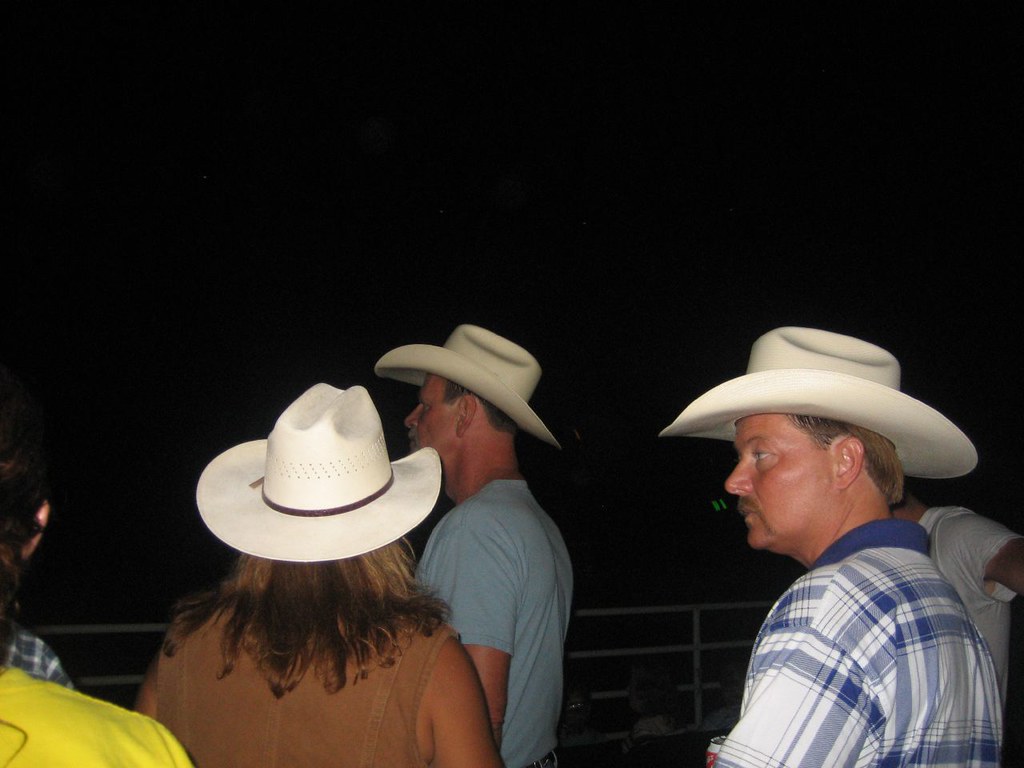In this nighttime photograph, set against a pitch-black background, we see a group of five people, though the image centers around three individuals who stand out due to the camera's flash. All of them are adorned in white Stetson cowboy hats, each featuring a brown border. The woman, positioned with her back to the camera on the left side, has long brown hair cascading past her shoulders and wears a sleeveless brown top. To her right, a man in a light blue shirt, sporting short hair and a mustache, stands slightly ahead. Adjacent to him is another man in a blue plaid shirt, looking towards the left. The partial view of individuals on the far left and far right shows one person in a white T-shirt and another in a yellow T-shirt, but their faces are obscured. A dimly visible silver fence lines the bottom part of the image, adding depth to the night scene wherein the trio seems to look outward, captivated by something in the unseen distance.